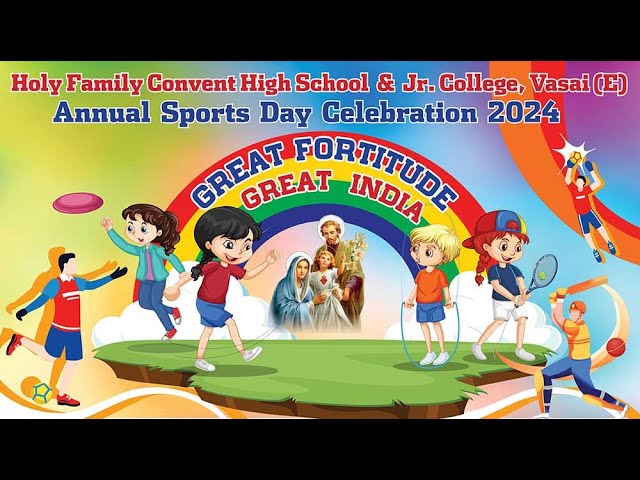This vibrant poster advertises the "Annual Sports Day Celebration 2024" for Holy Family Convent High School and Junior College, Sivasai (E). Depicting a radiant rainbow that spans the entire background in shades of red, yellow, green, and blue, the poster illustrates a lively scene with cartoon figures of children engaging in various sports, such as frisbee, soccer, jump rope, tennis, cricket, and basketball. At the top, bold red text declares the name of the school, while blue text just beneath announces the event. Atop the rainbow, the words "Great Fortitude, Great India" are prominently displayed. The overall design is decorated with a black border on the top and bottom, contributing to its striking visual appeal. The poster hints at a sense of community and vigor, inviting participation and emphasizing the importance of physical activity and resilience.